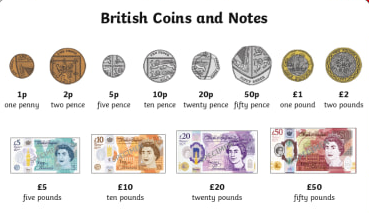The image depicts a comprehensive chart titled "British Coins and Notes" in bold black lettering at the top. It showcases various denominations of British currency, arranged in two rows. In the top row from left to right are the coins: 1 penny, 2 pence, 5 pence, 10 pence, 20 pence, 50 pence, 1 pound, and 2 pounds. The first two coins are brown, with the 1 penny being smaller than the 2 pence. The next two, 5 pence and 10 pence, are silver, with the 5 pence being smaller. The 20 pence and 50 pence coins are also silver but have distinct edges and are progressively larger. The 1 pound and 2 pound coins are silver with a yellow outline, with the 2 pound coin being slightly larger. The bottom row displays banknotes: 5 pounds, 10 pounds, 20 pounds, and 50 pounds, each featuring an image of the Queen and varied coloration—green, orange, purple, and a multicolor mix predominantly red, respectively. The notes increase in size with their value. The image also contains artifacts: a black dot in the upper left corner and a red triangle in the upper right corner, indicative of copying errors. This chart serves as an educational tool, possibly for classrooms or booths, aiding in the identification of British currency.